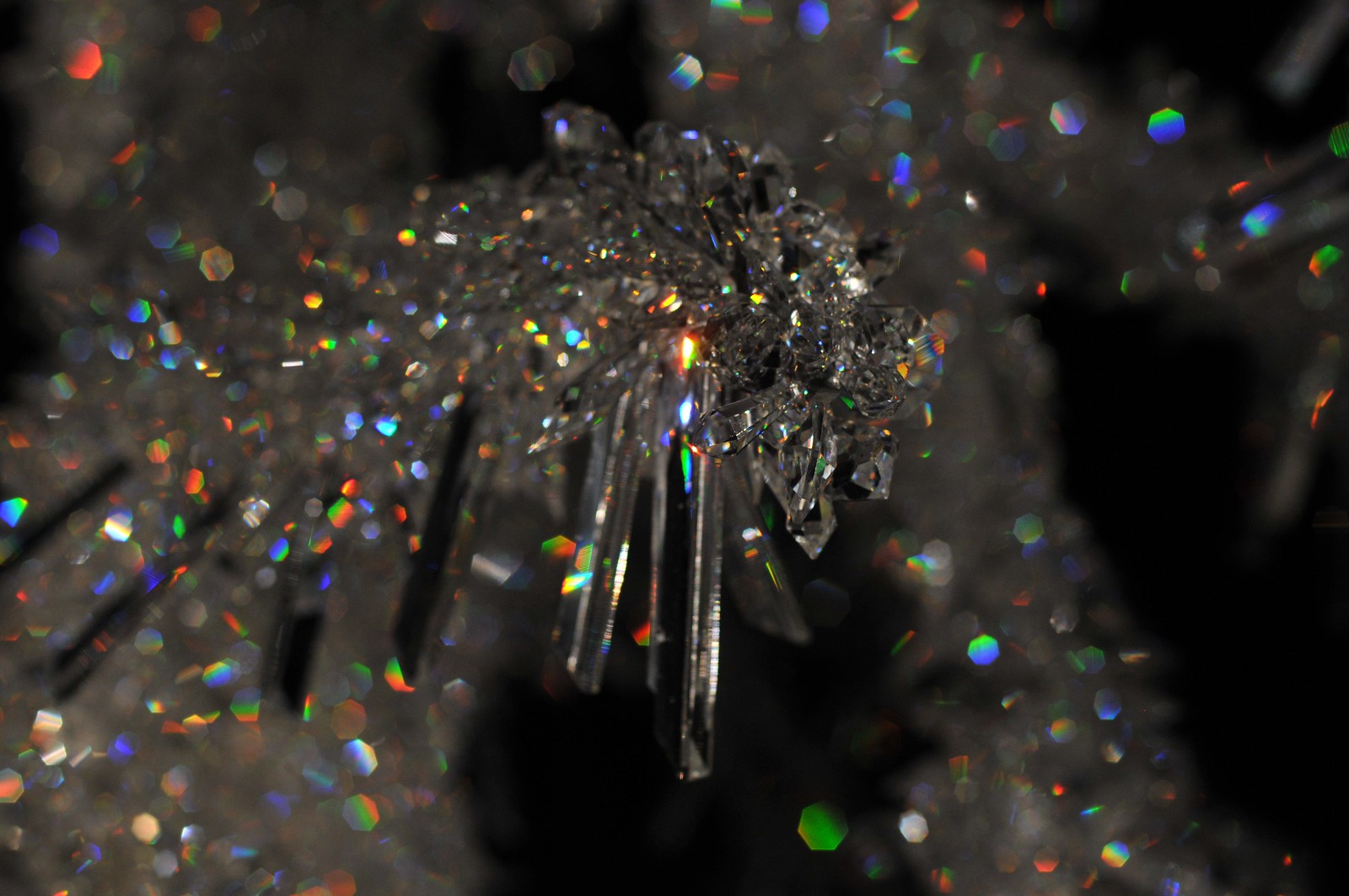This artistic photograph captures a close-up of what appears to be a fine crystal or possibly reflective tinsel, centrally positioned and in sharp focus. The crystal is surrounded by smaller, similarly reflective objects that create a blurred backdrop, enhancing the crystal's clarity and prominence. The interplay of light on the silver surface generates a multitude of prismatic colors, including reds, greens, blues, and whites, which are scattered throughout the image. These colors manifest as tiny, radiant dots, each with a mix of hues, enhancing the shimmering, glittery appearance of the scene. The overall setting is dark, possibly nighttime, which contrasts beautifully with the dazzling, light-reflecting crystal, creating a striking, multi-colored visual effect that combines elements of fractal light reflection and artistic depth. The image evokes a sense of wonder and beauty, reminiscent of holiday tinsel or a precious gemstone, captured in a landscape orientation.